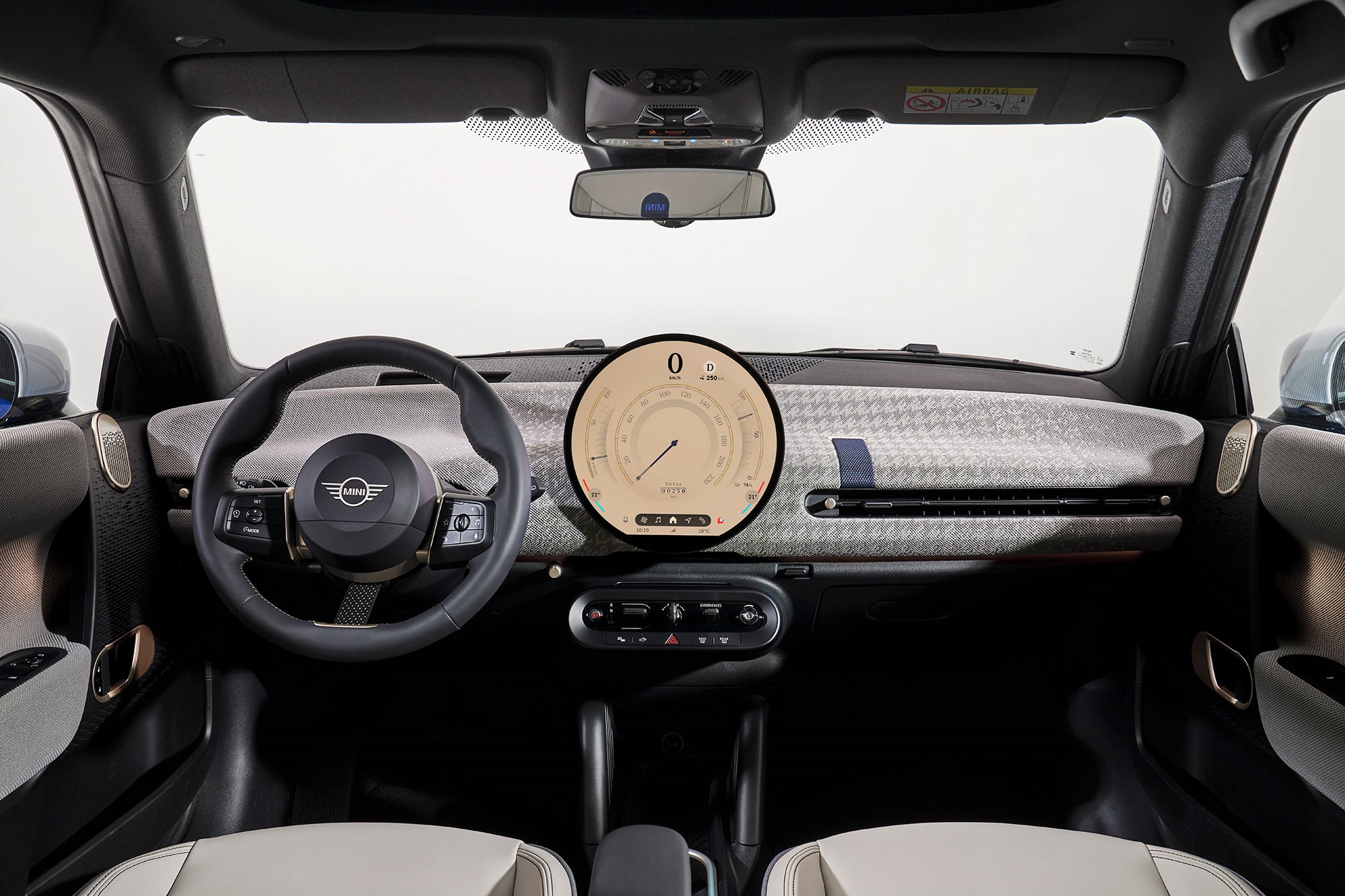This photograph, taken from the backseat of a compact vehicle, offers a clear view of the front interior. The minimalistic yet stylish design suggests a Mini Cooper, evident from the prominent circle and wing logo on the black steering wheel. The steering wheel is on the left, and the dashboard, adorned with a subtle decorative pattern, is primarily gray with a mix of black and light beige tones. The sizeable central speedometer, encased in a black-trimmed circular frame with a beige display, stands out against the sleek and simple dash, which also features the AC and heater controls. Light beige seats, only partially visible from this angle, add to the car's clean and uncluttered aesthetic. Through the front windshield and side windows, the outside scene is completely white, emphasizing the car's interior details and framing it as a product shot devoid of distractions.